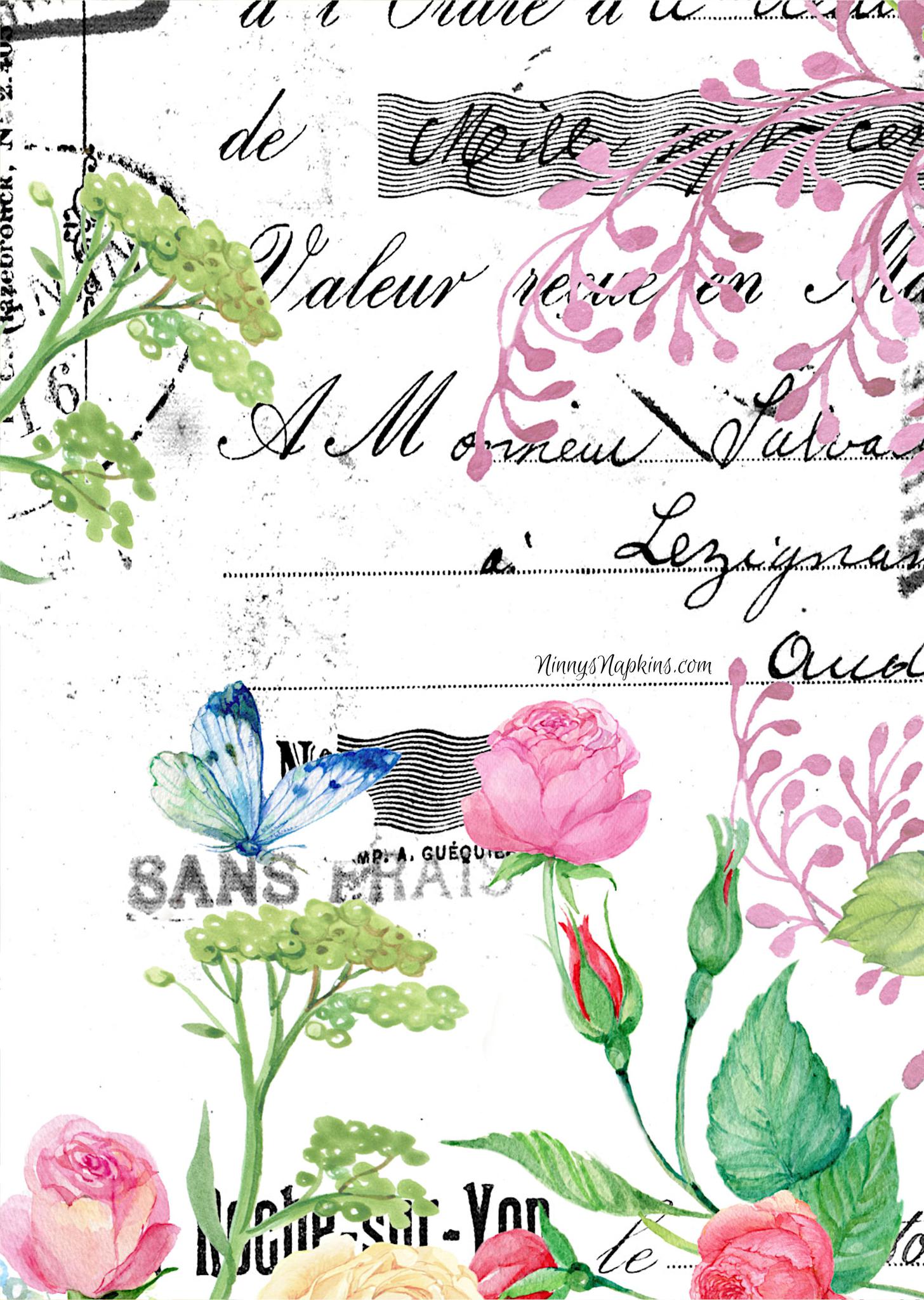The image showcases a delicate design resembling a card or possibly a napkin, with an all-white background akin to a pristine sheet of paper. Adorning this backdrop are intricate floral patterns featuring vibrant pink roses and partially blooming red rosebuds. In the top left corner, there's a lush green plant that bears a striking resemblance to a head of broccoli. Near the bottom, a graceful blue butterfly hovers, poised as if about to land on a plant. Elegant black cursive writing, seemingly in a foreign language, adds a touch of sophistication. Additionally, a small section of the design includes the text "NinniesNapkins.com," suggesting that this beautiful artwork is part of a purchasable napkin design from the mentioned website.